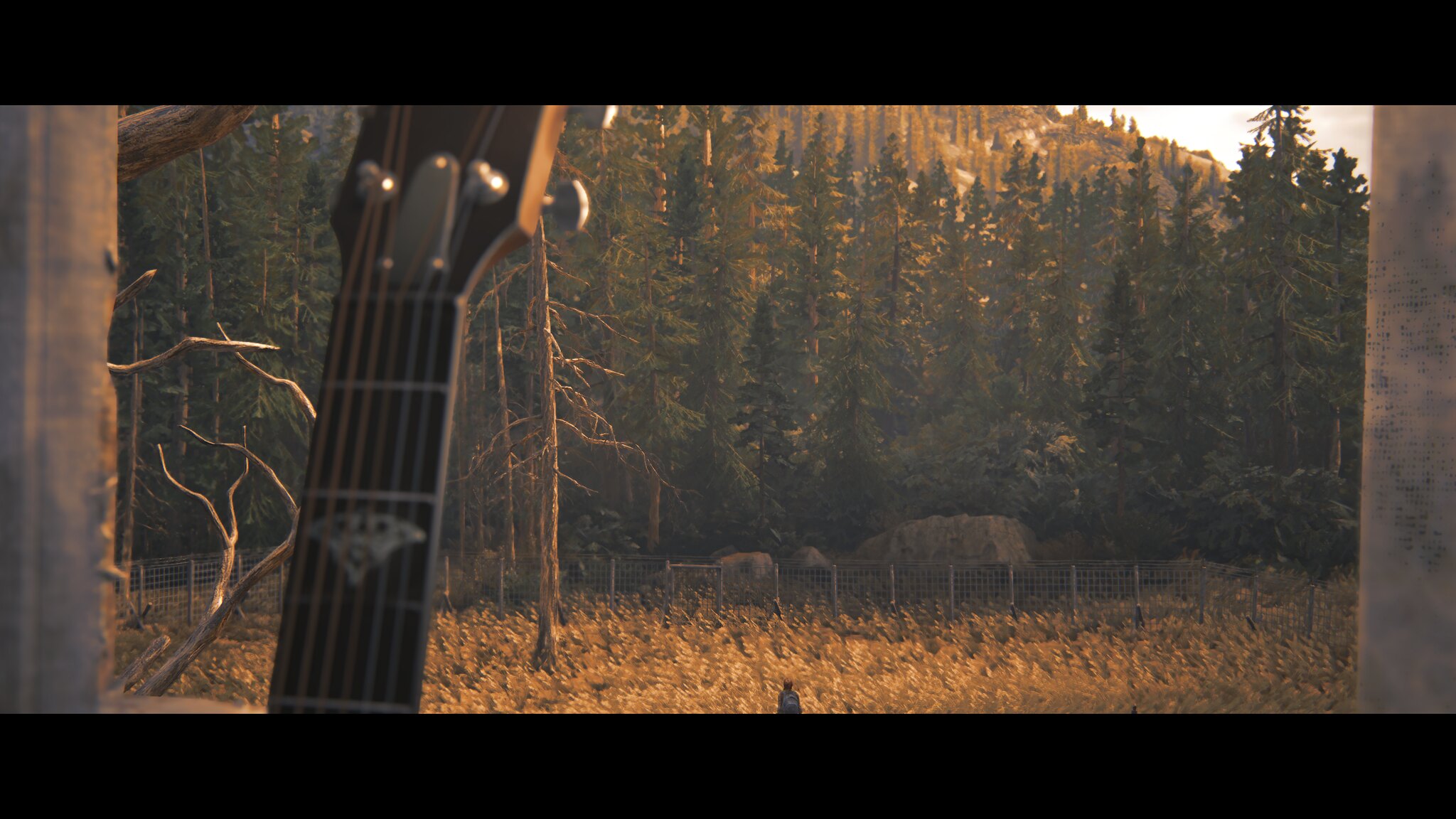The image captures a serene and expansive outdoor scene, showcasing a sectioned field bordered by a fence with an extensive forest in the background. Tall, lush green trees, resembling pine trees, rise majestically and extend towards rolling hills or mountains. Inside the fenced area, there are brownish patches that seem indicative of wheat or another type of crop. Scattered within the field are a few trees devoid of leaves, contrasting with their verdant counterparts further beyond the fence. A person appears small and distant, walking through the lower part of the field, adding a sense of scale to the vast landscape. In the immediate foreground, occupying a prominent place in the composition, is a close-up shot of the neck of a guitar, capturing about four frets and the tuning pegs. This convergence of natural elements and the musical instrument creates a tranquil and evocative scene. The overall palette of the image includes rich greens, browns, and subtle grayish tones from the rocks near the fence, enhancing the peaceful ambiance.